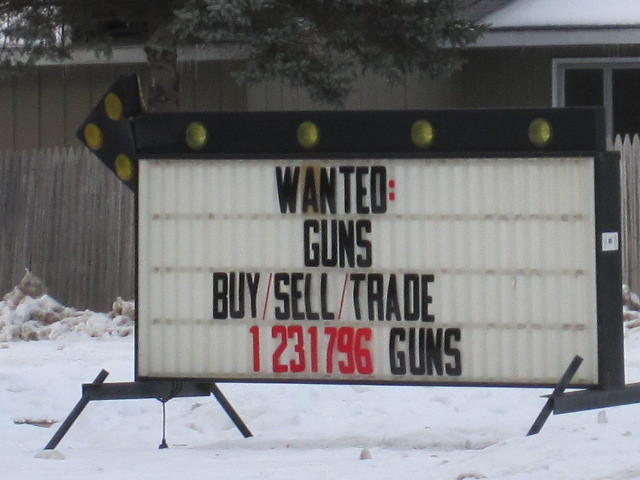The photograph features a prominent black metallic marquee sign sitting in the snow on the ground. The sign, which probably can light up despite currently being unlit, has a large arrow on top pointing to the left. The arrow is decorated with yellow lights inside. The sign has a white background with black, easily changeable letters spelling out "WANTED GUNS. BUY, SELL, TRADE." The phone number "1-2-3-1-7-9-6" is written in red, followed by the word "GUNS" in black letters below it. Surrounding the sign is somewhat dirty snow, indicating the area has been trodden on. In the background, there is a wooden house or cabin surrounded by a wooden fence, partially obscured by foliage from a tree overhead that has no snow on it. The house appears grayish in color and gives the impression of being in a residential area.